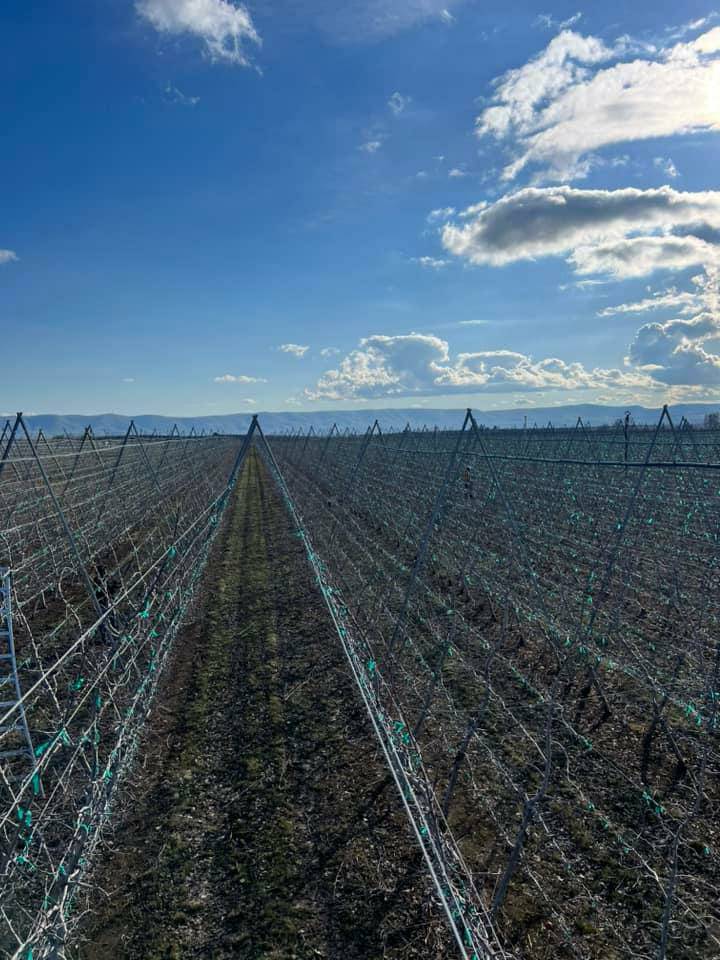In this detailed photograph of a rural farm field, the ground is covered in a mix of brown and green soil, arranged in vertical sowing lines. The field is lined with sharp, metallic wire fences that extend toward the horizon, flanked on both sides and gradually diminishing from view. These fences are designed to protect the young plants, which are yet to sprout fully, and some have green leaves or vines creeping up them. Additionally, there are triangular wooden structures placed over sections of the field for further plant protection, though the center of these structures reveals empty, tilled soil. Above, the sky is a clear blue with a mix of white and gray clouds mostly scattered to the right side of the image. The sunlight, indicative of a mid-afternoon setting, illuminates the landscape from the right. In the far background, beyond the edge of the field, gentle hills complete the serene rural scene.